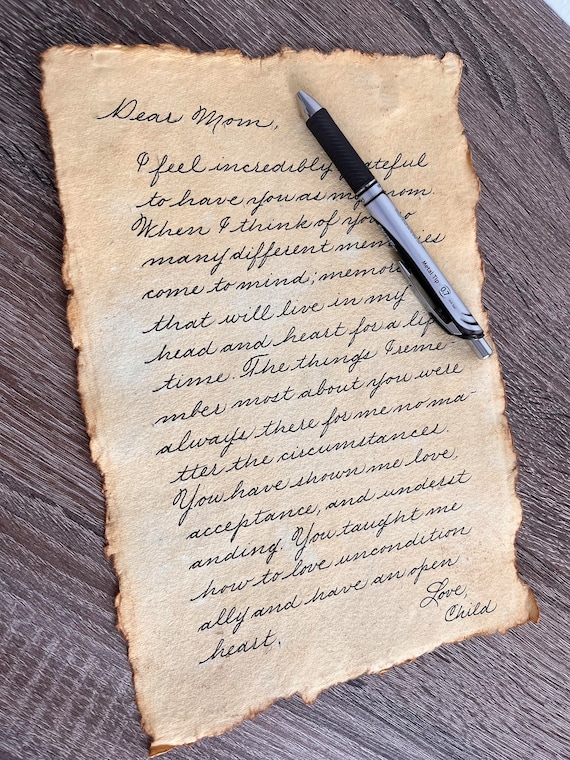This color photo, shot from above, captures an antique letter on an aged, tan brown sheet of parchment paper, placed on a dark brown, heavy-grain wooden table. The letter, which appears worn with burnt, brownish, orangey-red edges, starts with "Dear Mom" and ends with "Love Child." Penned in elegant cursive, the letter expresses deep gratitude and love, mentioning cherished memories and values such as unconditional love and open-heartedness. A gray mechanical pencil or pen with a black grip rests at the top right corner of the letter, partially obscuring some of the heartfelt text.